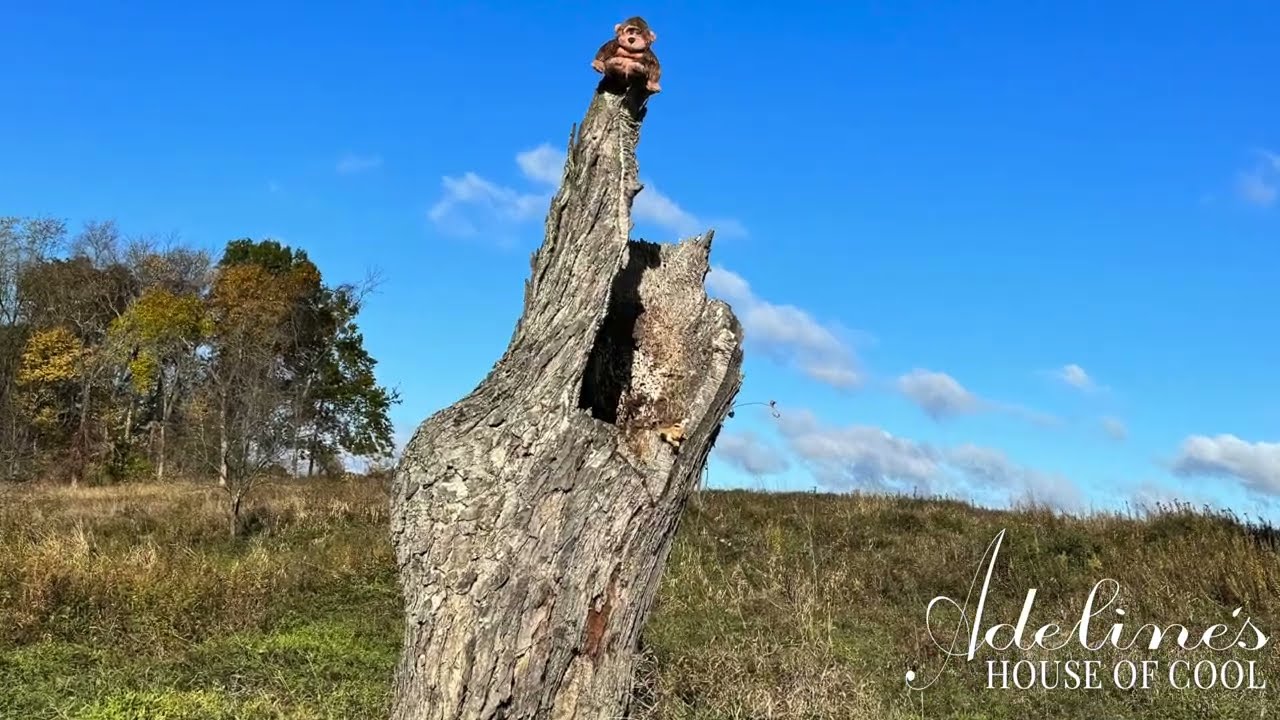This horizontal photograph captures a relatively wild outdoor scene under a bright blue sky with a few scattered white clouds. Dominating the center is a striking, almost dead tree stump, white and gray in color, with a jagged top that looks like it was snapped off. Perched at the peak of this broken trunk is a brown stuffed animal, which closely resembles a monkey with a black nose and tan face, belly, and paws. Surrounding the tree stump is a field of unkempt, weedy grass, adding to the natural, untamed ambiance of the setting. To the left and in the background, a cluster of tall, green and yellow trees rise up, contributing to the sense of being in a secluded nature spot. The image also includes some subtle textual elements; in the bottom right corner, scripted in white text, it reads "Adeline's," followed by "House of Cool" in all capital letters.